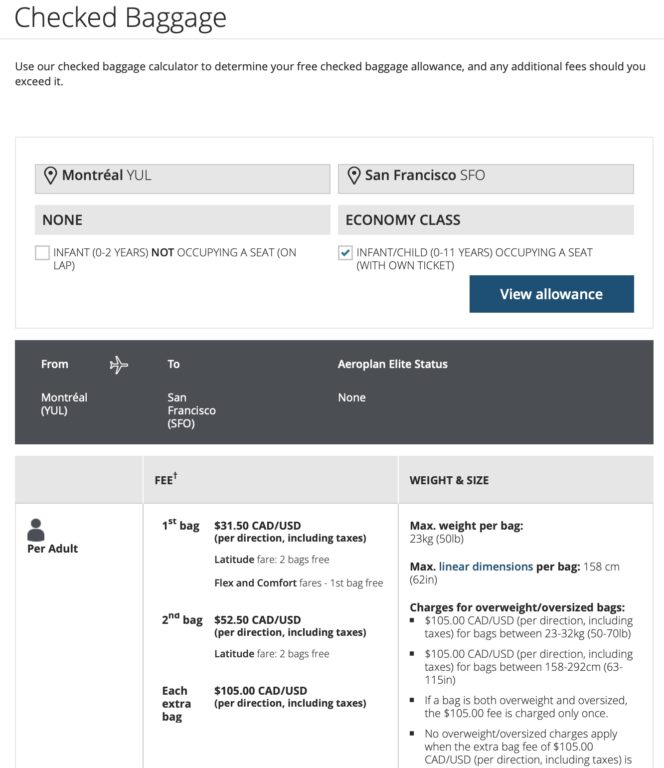Screenshot of a Checked Baggage Web Page

Detailed Description:

This screenshot captures a web page for calculating checked baggage allowances. The interface is primarily white with black text. In the upper left corner, the title reads "Checked Baggage," instructing users to utilize the checked baggage calculator to determine their free checked baggage allowance and any additional fees for exceeding it. 

The journey details are specified as follows:
- Departure: Montreal, YUL
- Arrival: San Francisco, SFO

For class selections, one option indicates "Economy Class," and another notes specific allowances for different types of passengers:
- Infant (under 2 years) not occupying a seat, held on lap.
- Child aged 0-10 years with an individual seat and own ticket.

There is a prominent blue button with white lettering that says "View Allowance."

Below this, encased in a gray box, are additional travel details, reiterating:
- From: Montreal, YUL
- To: San Francisco, SFO

It also includes specifics for fare types and statuses:
- Aeroplan status: None
- Pricing details for various fare types appear at the bottom, detailing checked baggage fees:

  - Per adult: 1 bag is $31.50 CAD or USD per direction, including taxes.
  - Latitude fare: 2 bags are free.
  - Flex and Comfort fares: The first bag is free, and the second bag costs $50.50 CAD or USD per direction, including taxes.
  - Latitude fare: Each extra bag is $105 CAD or USD per direction, including taxes.

Additional baggage details:
- Maximum weight per bag: 50 pounds.
- Maximum linear dimensions: 158 centimeters or 60 inches.
- Multiple charges are listed for overweight and oversized baggage.

The overall impression is that numerous additional fees apply for excess or oversized baggage, emphasizing the financial burden on travelers for extra luggage.